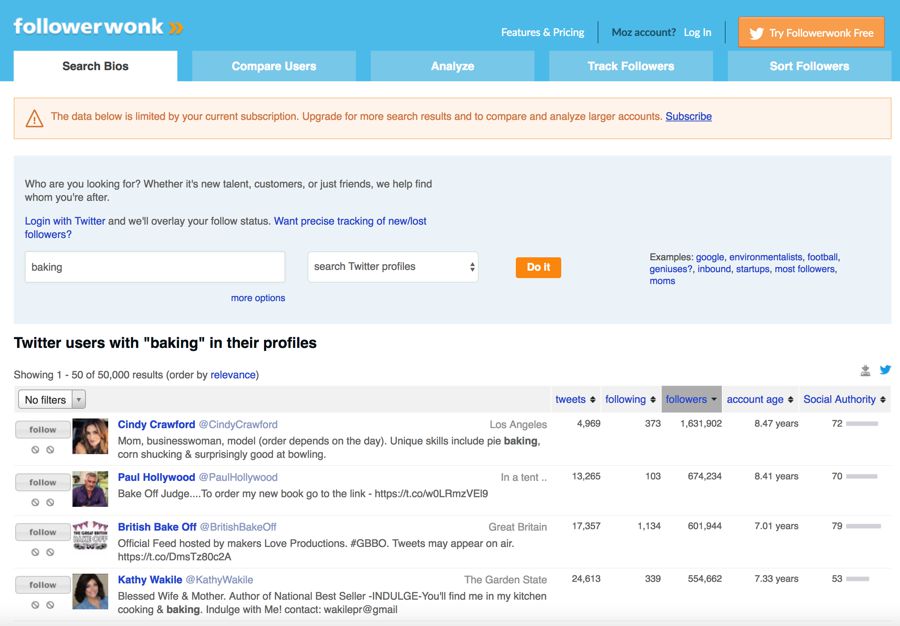A screenshot from a website's search area features prominently in the image. In the top left corner, the text "Follower Walk" is displayed. The interface indicates that the user is currently in the "Search Files" section. A notification is situated beneath the header, stating: "The data below is limited by our current subscription. Upgrade for more search results and to compare and analyze larger accounts."

In the search box, the term "baking" has been entered. Below the search bar, there is a heading that reads: "Twitter users with 'baking' in their profile." The search results list is displayed, starting with "Cindy Crawford," followed by "Paul Hollywood," "British Bake Off," and the final entry, "Kathy Ligwaki." The detailed yet concise layout provides a clear view of how users with interests in baking are being queried and presented on this platform.